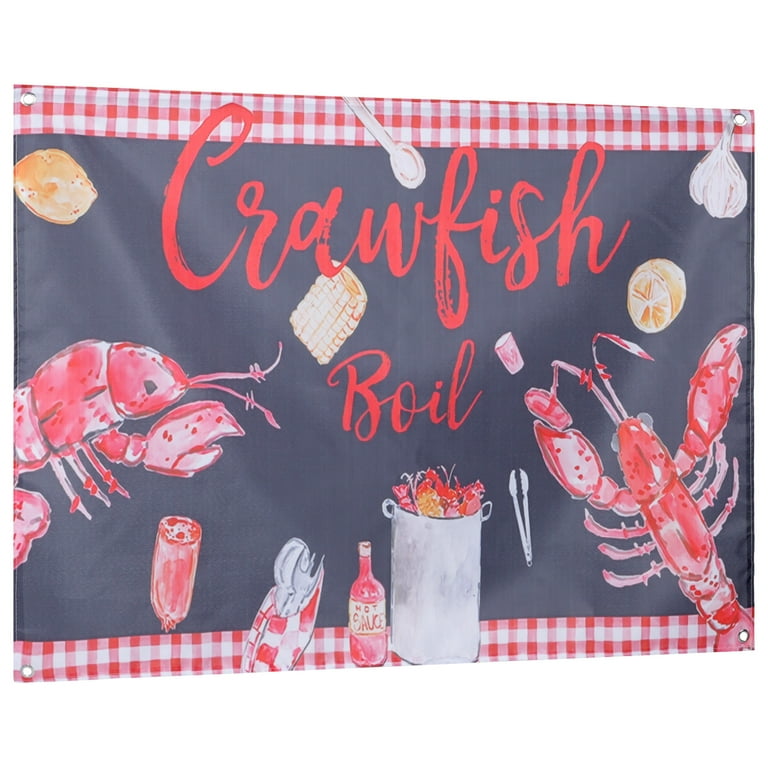The image is an advertisement for a crawfish boil, designed with a classic red and white checkerboard pattern at the top and bottom borders, reminiscent of a picnic tablecloth or flag. The central background is black, and prominently features the phrase "Crawfish Boil" in elegant, large red cursive script at the top center. The image is filled with elements typically associated with a crawfish boil, including crawfish, lobsters, corn on the cob, what appears to be buttered rolls or biscuits, and garlic. A variety of utensils are scattered throughout the image, such as forks, spoons, tongs, a larger spoon at the top middle, and a spoon and fork wrapped in a napkin. There are also condiments depicted, including a bottle of Tabasco sauce and what looks like ketchup. Additionally, the image features other items like lemons, a pitcher filled with a red and yellow liquid, and some round slices that could be salami or similar food items. The overall setup gives the impression of a festive, well-stocked crawfish boil setting.